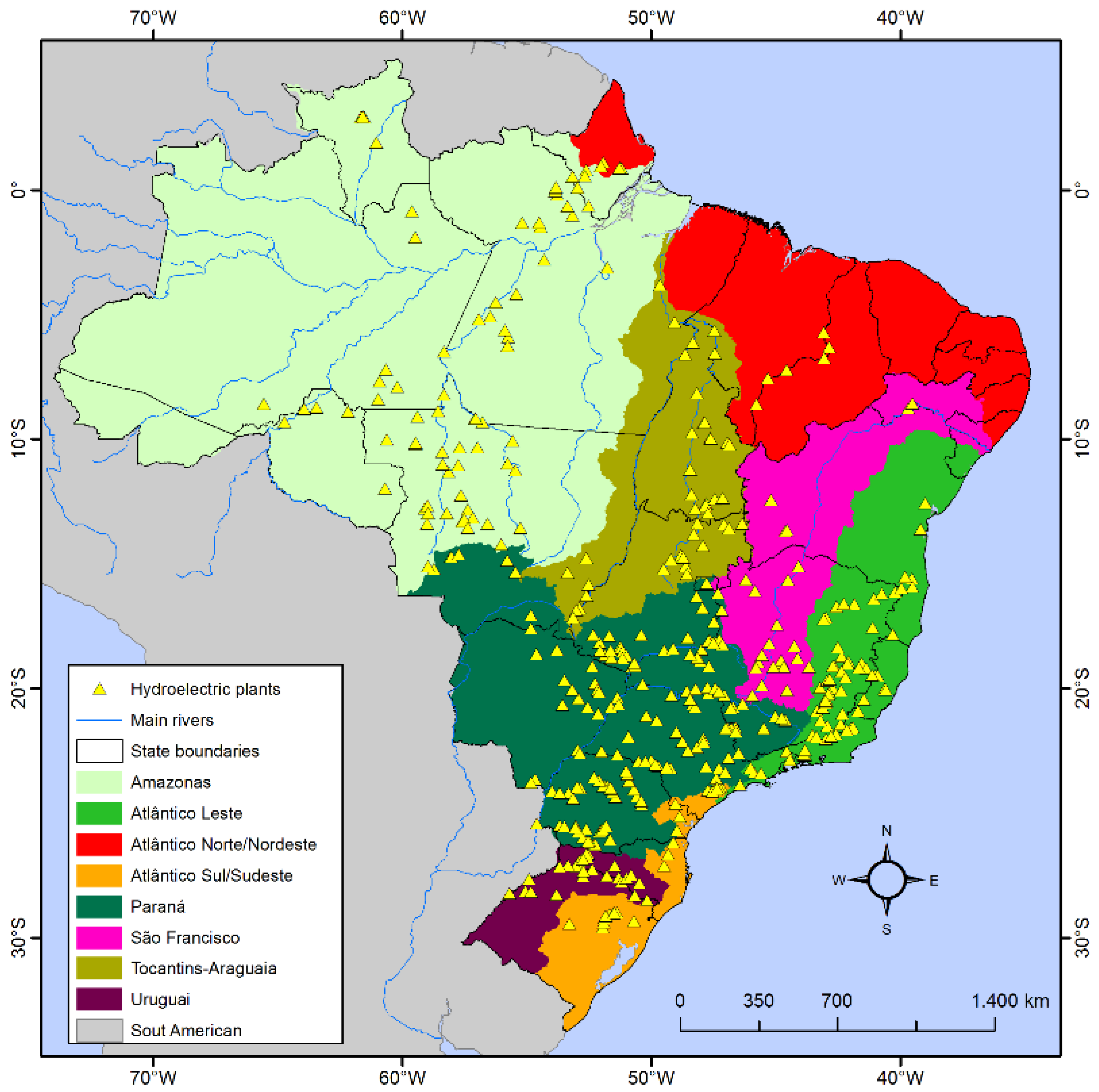This detailed geographic map of South America is color-coded to delineate various regions, which are prominently labeled in Spanish. The map encompasses predominantly Argentina and Brazil, with surrounding areas in gray. Each region is distinctively marked: light green for Amazonas, lime green for Atlantico-Leste, red for Atlantico-North, orange for Atlantico-South, dark green for Parana, hot pink for Sao Francisco, and olive green for Tocantins. The regions South America and Uruguay are also indicated. The map is adorned with blue lines representing rivers and yellow triangle symbols that identify hydroelectric plants throughout the map. A legend on the left side explains the color codes and symbols. The map includes degree markers, a compass for orientation, and a measurement scale in kilometers, with all latitude and longitude lines marked in degrees, providing detailed navigational information.